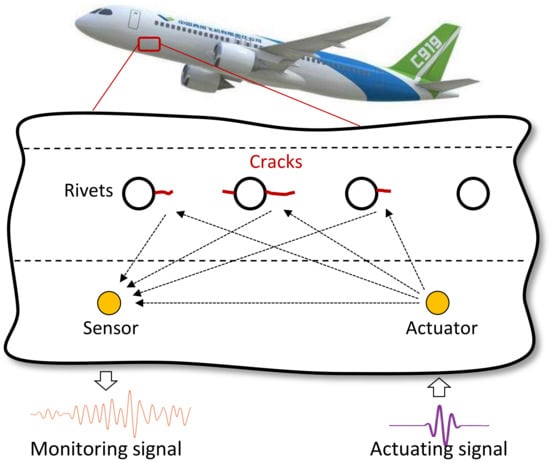The image is an infographic of a passenger airplane, the C919, set against a solid white background. The airplane at the top of the diagram is white with a blue stripe on the back end and a green fin, prominently labeled "C919." Below the airplane is a detailed chart pointing to various technical aspects of the aircraft's side, including cracks, rivets, sensors, and actuators. The chart features clear circles and black arrows indicating the locations of these elements on the front lower section of the plane. Additionally, there are terms such as "monitoring signal" and "actuating signal" displayed underneath the diagram, accompanied by graphical arrows and wave signals, all of which seem to emphasize the inspection and monitoring points of the aircraft's hull.